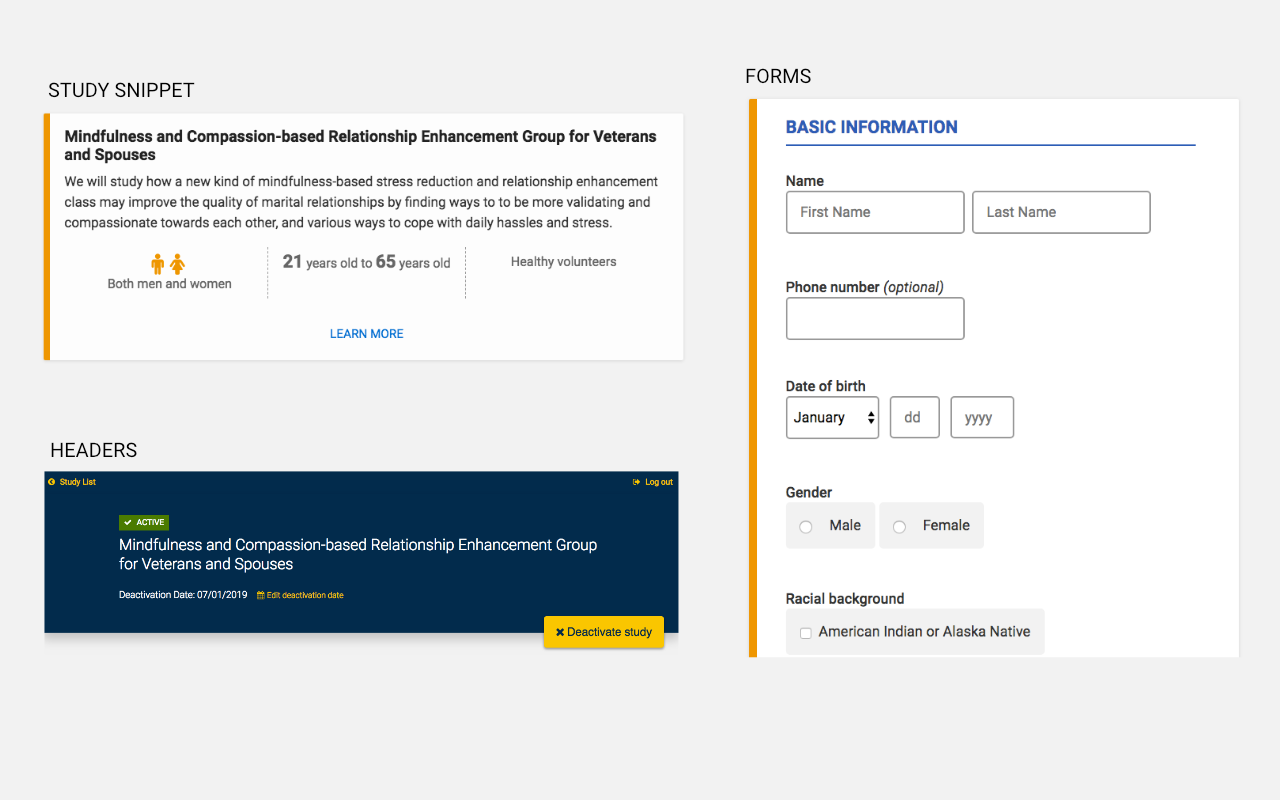The image depicts a webpage with the header "Study Snippet," focused on a program titled "Mindfulness and Compassion-Based Relationship Enhancement Group for Veterans and Spouses." The webpage details a study aimed at evaluating how a novel mindfulness-based stress reduction and relationship enhancement class can improve marital relationships by promoting validation, compassion, and effective coping strategies for daily stressors. 

At the top of the page, an icon indicates the study is open to both men and women aged 21 to 65 years, targeting healthy volunteers. Below this section, there's a blue 'Learn More' button. 

Underneath various headers, there is a section labeled "study list" with the title "Active Mindfulness and Compassion-Based Relationship Enhancement Group for Veterans and Spouses." The deactivation date for the study is listed as July 1, 2019, with an option to edit this date or deactivate the study, highlighted in yellow. 

A logout button is situated in the top corner. 

The "Forms" section offers fields for basic information, including first name, last name, and an optional phone number, along with fields for date of birth divided into month, day, and year. Gender options are provided as male and female, and there is an additional option to specify racial background.

The webpage's design features a gray background, with white input boxes and black text for clear readability.